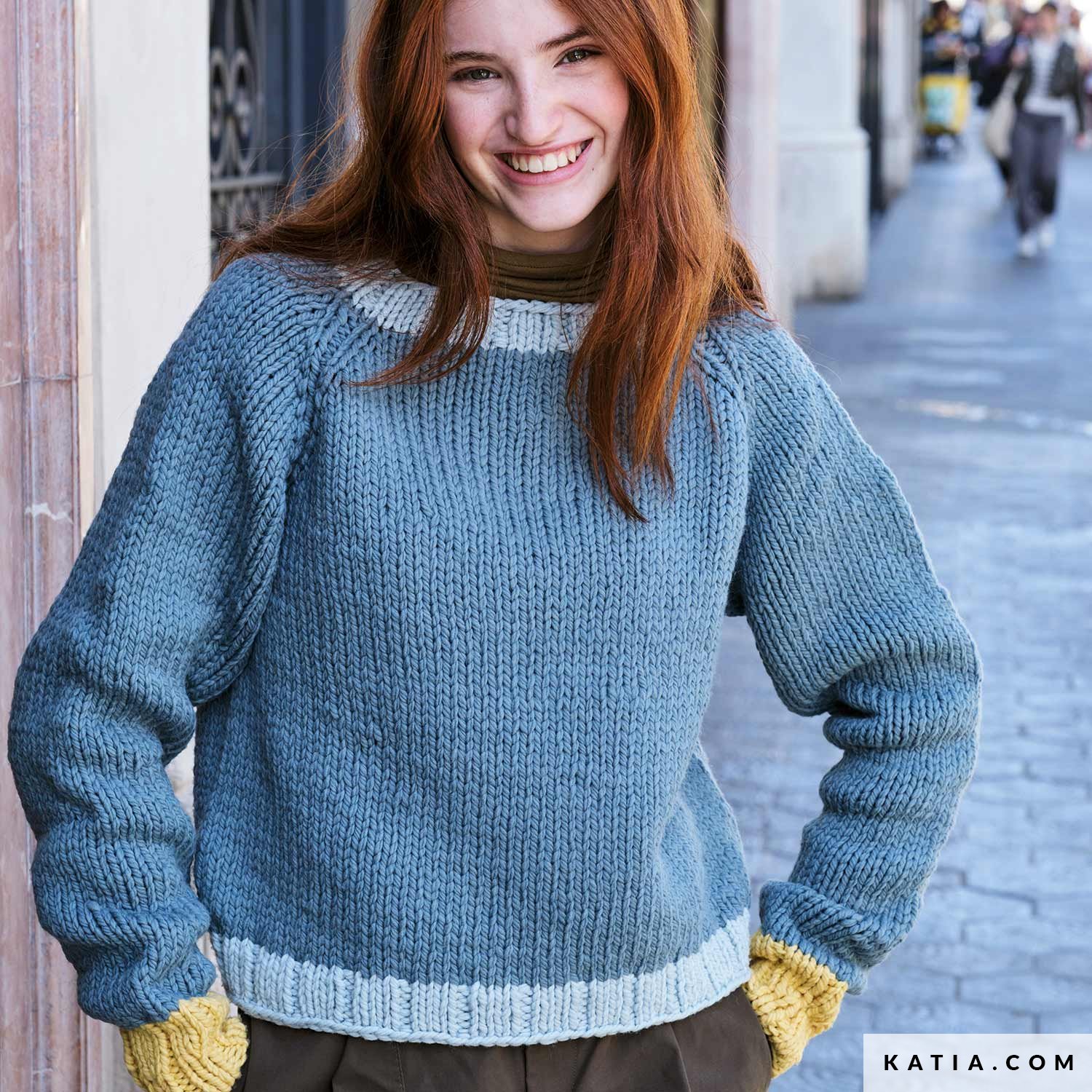The advertisement features a close-up image of a woman with red hair that extends below her shoulders and brown eyes, smiling brightly at the camera. She is wearing a bulky, knitted blue sweater with several accented colors: a light sky blue neckline, matching light blue bands at the bottom hem, and yellow wrist cuffs. Her hands are tucked into the sweater's pockets, concealing them. She pairs the sweater with brown pants. In the background, there's a cobbled city sidewalk and a blurred building, adding depth to the scene. Distant, out-of-focus figures can be seen walking along the sidewalk. In the bottom right corner of the image, the text "K-A-T-I-A dot com" is prominently displayed.